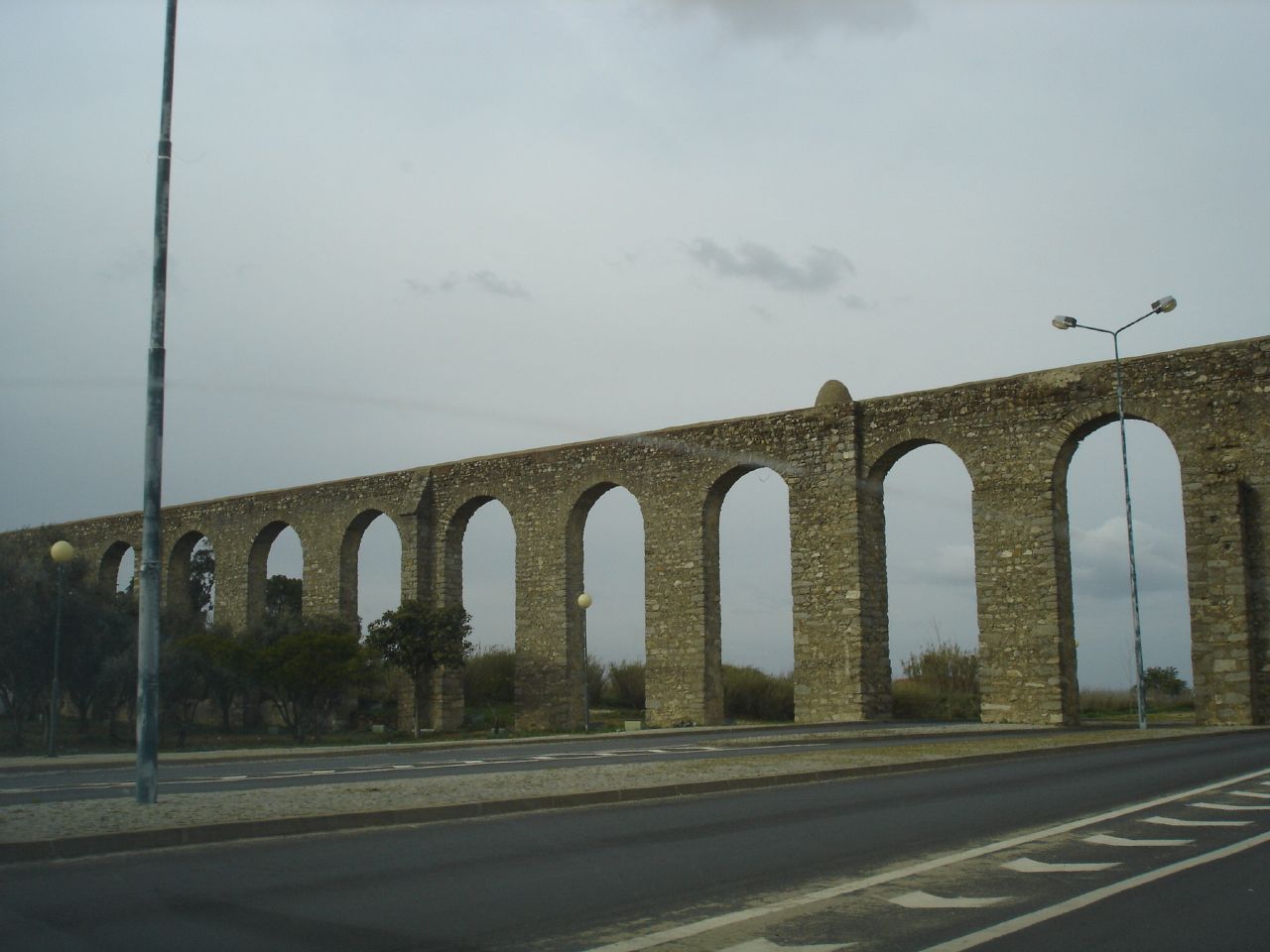The image captures a gloomy, overcast day featuring a cobblestone bridge with multiple stone and brick arches stretching across a two-lane roadway. The road, marked by white stripes, passes beneath the weathered archways of the bridge in a median that has tall, silver streetlight poles, each adorned with lights pointing in both directions. On the left side of the image, in front of the bridge, there's a small patch of green trees, while on the far side of the bridge, smaller, brownish trees are visible. The aged and darkened appearance of the bridge, coupled with the cloudy, gray sky, suggests recent rain, adding to the overall somber atmosphere. Directional arrows on the road guide vehicles to ensure correct traffic flow.